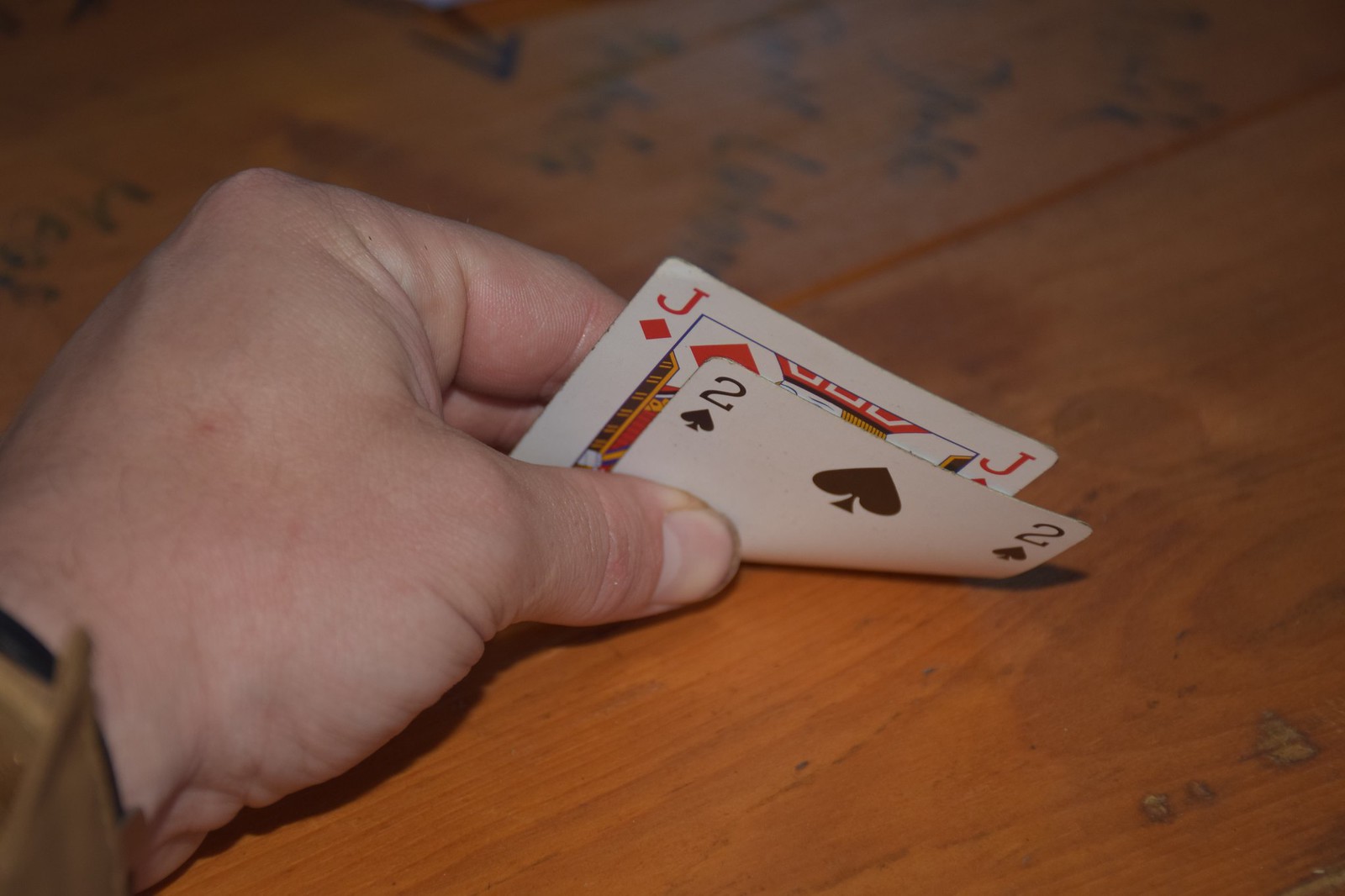A detailed photograph captures the rustic charm of a brown wooden table composed of distinct planks, each marked with linear patterns. Faint, blurry text in black appears at the top of the table. From the bottom left corner, a hand, presumably of a Caucasian individual, extends onto the table. The wrist is adorned with a brown accessory beneath a black one. The person's thumb, featuring a somewhat elongated and dirty fingernail, holds two playing cards. The cards are slightly curled at their ends. The visible cards are the two of spades, lying directly on the table, and behind it, partially visible, is the jack of diamonds. Subtle shadows of the cards add depth to the image.